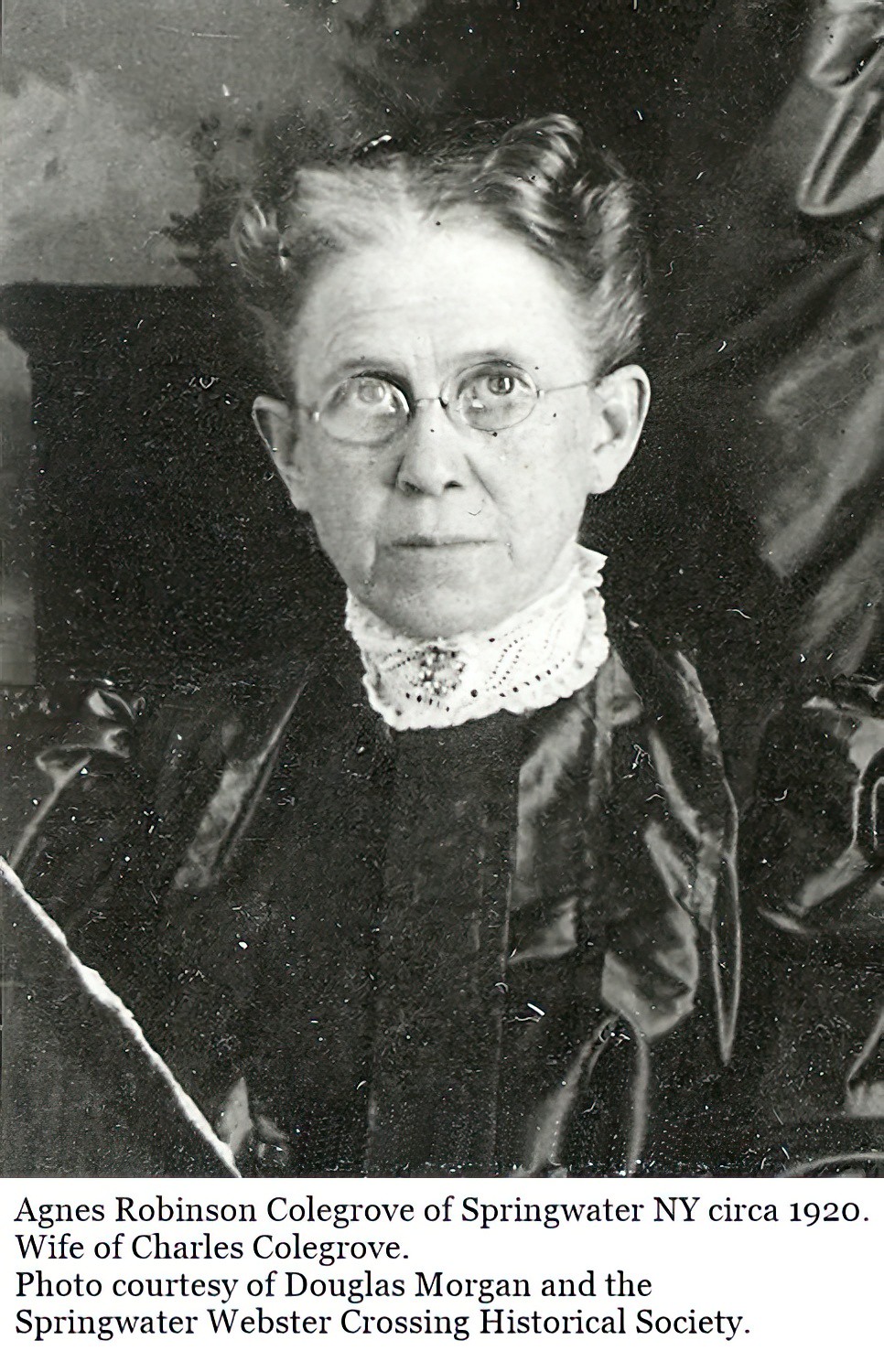This black-and-white photograph, taken circa 1920, shows an elderly woman named Agnes Robinson Colgrove of Springwater, New York. She is depicted from the chest up, set against a dark background. Agnes gazes directly at the camera with a serious expression. Her gray hair, parted down the center, is gathered and secured, possibly with a clip or barrette, on top of her head. She wears round, wire-rimmed glasses and a distinctive white lace collar, adorned with a brooch at the center. Her attire features a black, shiny top with puffy, long sleeves and black buttons running down the front. The caption underneath the image reads: "Agnes Robinson Colgrove of Springwater, N.Y., circa 1920, wife of Charles Colgrove. Photo courtesy of Douglas Morgan and the Springwater-Webster Crossing Historical Society."